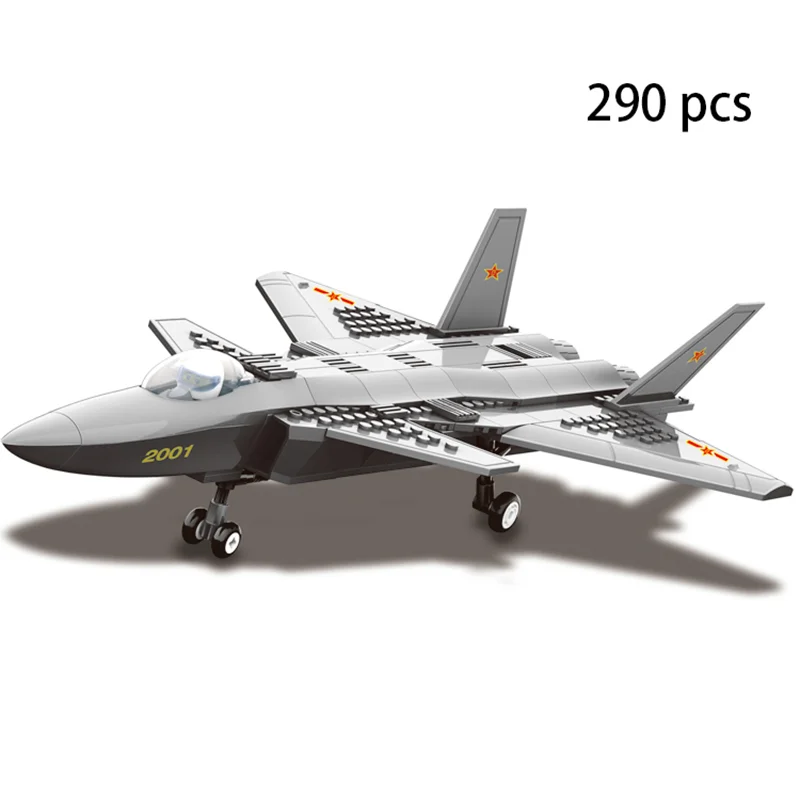This image depicts a detailed, 290-piece fighter jet model constructed from Lego-type blocks. The jet, built with a combination of light grey and dark grey blocks, is displayed on a stark white background with a subtle shadow cast beneath it. Prominently, "2001" is labeled at the nose of the aircraft, with orange stars marked on the back fins. The model features two wheels in the front and intricate details like the notches for piece connection on the top wings. The cockpit houses a small, faceless, helmeted figure enclosed in a glass dome. The numerical "290" alongside the lowercase text "pecs" is positioned at the top right of the image, complementing the detailed visual of this Lego fighter jet model.